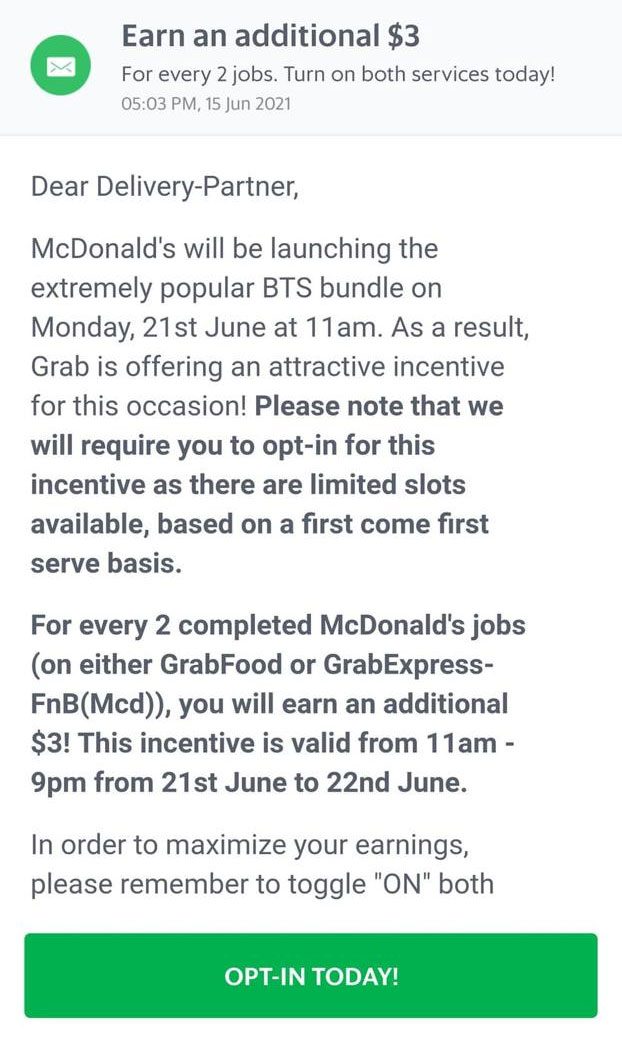A screenshot showcases a notification seemingly from an email or gig work platform. At the top, bold text announces an incentive: "Earn an additional $3 for every two jobs, turn on both services today." Dated 5:03 PM June 15th, 2021, the message greets "Dear Delivery Partner" and proceeds to inform about McDonald's upcoming BTS Bundle launch on Monday, June 21st at 11 AM. 

The communication details an enticing offer from Grab, presenting a chance to earn extra by completing McDonald's delivery jobs. The incentive requires opting-in due to limited slots on a first-come-first-served basis. Specifically, for every two completed jobs via either Grab Food or Grab Express F&B MCD, an additional $3 will be rewarded. The promotional period is valid from June 21st to June 22nd, between 11 AM to 9 PM. 

To optimize earnings, drivers are encouraged to activate both services. Prominently displayed at the bottom is a green button labeled "Opt-In Today" in white text, inviting immediate action.